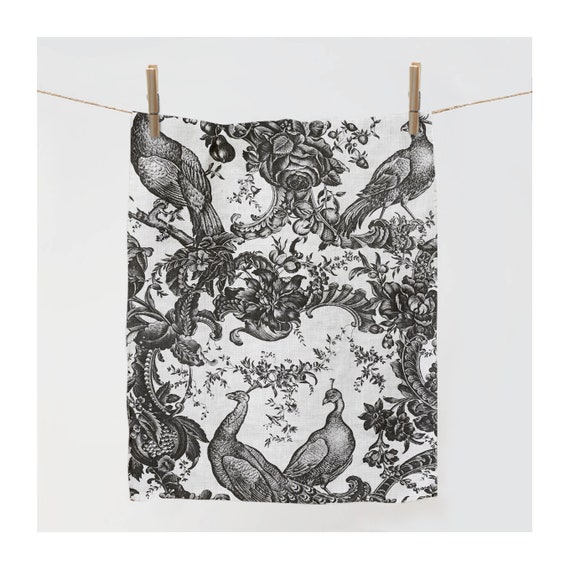This image captures a detailed, hand-drawn, black-and-white tapestry suspended by two hangers on a thin, light brown rope against an eggshell-colored wall. The tapestry showcases an intricate Victorian-era print resembling historic wallpaper, meticulously shaded without any color. The scene depicts four birds, likely peacocks, strategically placed—two perched at the top and two situated on the ground below. These birds are surrounded by a rich array of foliage including multiple flowers, such as roses and possibly snapdragons, with leaves extending gracefully from the sides. The attention to detail in the botanical elements and the birds' varied poses creates a textured, timeless aesthetic.